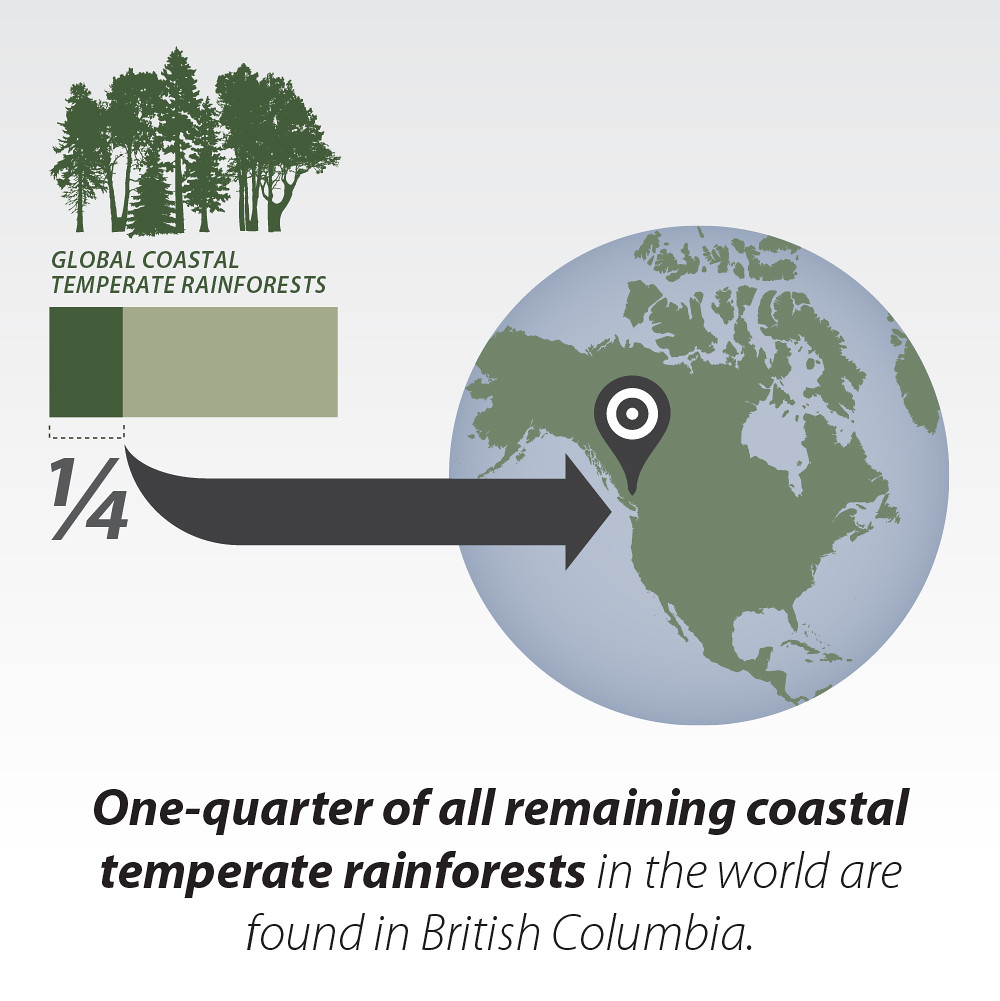The poster starts with a gradient background transitioning from gray at the top to white at the bottom. At the top, there's a silhouette of leafy trees and a pine tree. Below the trees, in green lettering, it reads "Global Coastal Temperate Rainforest." Underneath, a rectangular bar begins with a dark green left portion comprising one-fourth of the bar, and the rest in gray. Below the bar, the fraction "1/4" is displayed. An arrow extends rightward from the bar, pointing toward the center of an Earth image that features light blue oceans and gray landmasses. The arrow targets a bullseye near the California area, specifically aimed at the west coast of Canada. Below this, in gray lettering, it states, "One quarter of all remaining coastal temperate rainforests in the world are found in British Columbia."